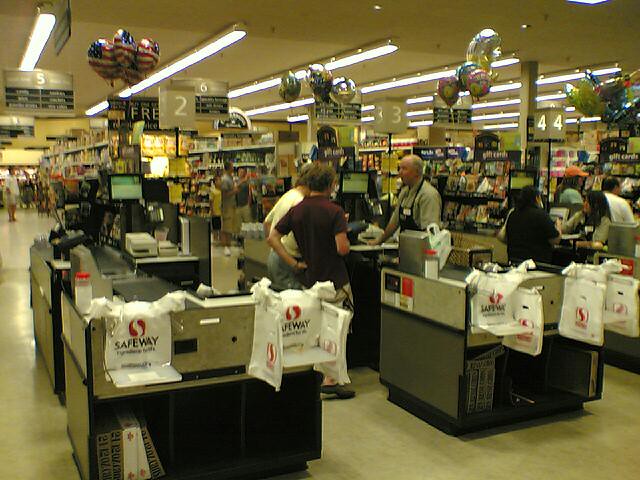This image captures the bustling checkout area of a Safeway supermarket from behind the cashier's stations. Two prominent cashier stations, labeled as lines 3 and 4, dominate the foreground, while a third station is partially visible in the background to the right. At the center of the image, between lines 3 and 4, a checker, identifiable by a black apron and gray shirt, assists two customers; one clad in a maroon shirt and the other in white. The checker at line 4 is also in uniform, tending to another customer dressed in black. The signature Safeway plastic bags, sporting a white 'S' on a red background, prominently hang at the end of each station. 

In the backdrop, several store aisles are visible, alongside hanging signs indicating aisle numbers and contents. The image includes aisles 2, 5, and 6, with additional shoppers seen throughout, including a parent with two children in aisle 2. American flag-themed balloons float at the upper left corner, accompanied by clusters of other colored balloons—pink, yellow, green—moving towards the right. The entire scene is bathed in a yellowish hue, adding a warm tone to the busy supermarket setting.